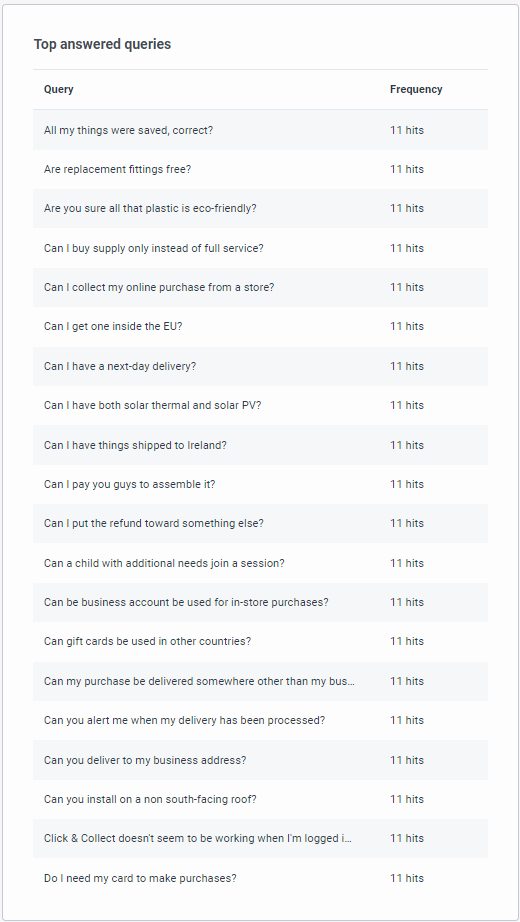This is a detailed caption for the given image:

"Screenshot with a white background displaying a table of top answer queries, sorted by frequency. Each query in the list has a frequency of 11 hits. The queries include: ‘Are all my things saved correctly?’, ‘Are replacement fittings true/free?’, ‘Are you sure all that plastic is eco-friendly?’, ‘Can I buy supply-only instead of full service?’, ‘Can I collect my online purchase from a store?’, ‘Can I get one inside the EU?’, ‘Can I have next day delivery?’, ‘Can I have both solar thermal and solar PV?’, ‘Can I have things shipped to Ireland?’, ‘Can I pay you guys to assemble it?’, ‘Can I put the refund towards something else?’, ‘Can a child with additional needs join a session?’, ‘Can the business account be used for in-store purchases?’, ‘Can gift cards be used in other countries?’, and ‘Can my purchase be delivered somewhere other than my business?’. The list emphasizes the diverse inquiries users have regarding product services and delivery options."